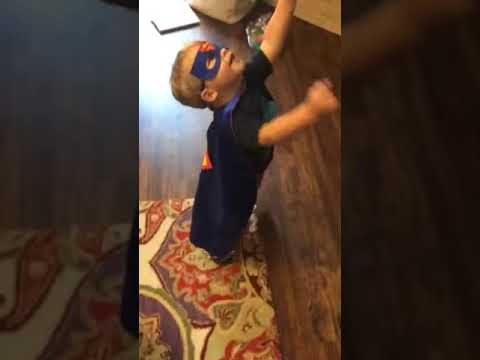Indoors, a young child stands on a multi-colored rug that has beige, brown, red, and green hues, adorned with floral or squirrel patterns, against a darker wood floor. The child, positioned at the center of this vertical image, is dressed as a superhero in a dark t-shirt and a dark cloak, with a greenish-blue symbol partially visible on the chest. He wears a mask with eye cutouts and has short hair, visible right ear, and exposed nose and mouth. His arms are upstretched, with the left arm straight up and the right arm slightly curved, as he tilts his head back to look at the ceiling—creating a dynamic, triumphant pose. The upper portion of the image shows a snippet of an Ottoman chair or couch, and a piece of paper or book is situated in the upper left corner. Two vertical black bars frame the portrait, adding to the dramatic effect.